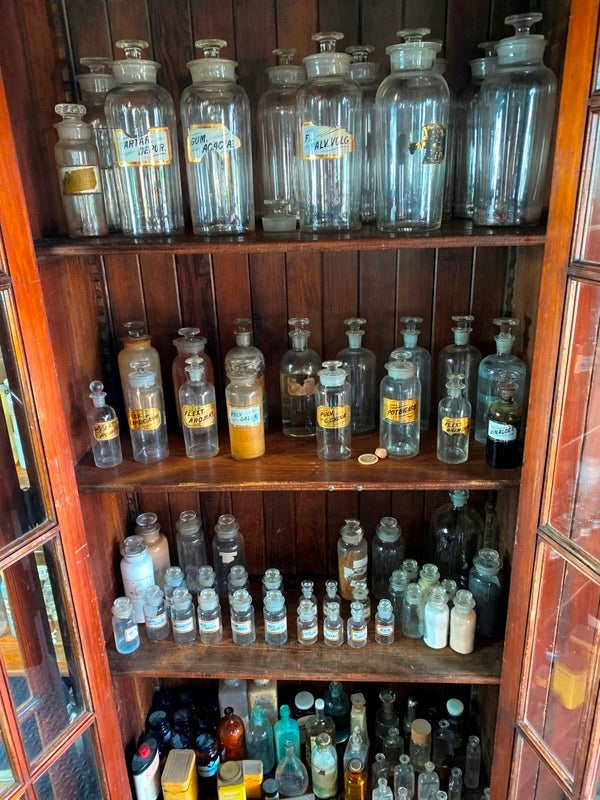In the image, an open wooden cabinet with glass-paneled doors reveals its contents across four shelves. The cabinet is predominantly brown, with varying shades throughout its structure. The top shelf holds the largest glass bottles, which are uniform in size and all empty, with some featuring labels. The second shelf contains a mix of bottles, some filled, including one with an orange liquid and another with a black liquid, and several with gold labels. The third shelf displays a variety of both larger and smaller bottles, some filled but mostly empty. The bottom shelf is the most diverse, showcasing a chaotic assortment of containers and canisters in different sizes and colors, including orange, yellow, brown, green, and gold.